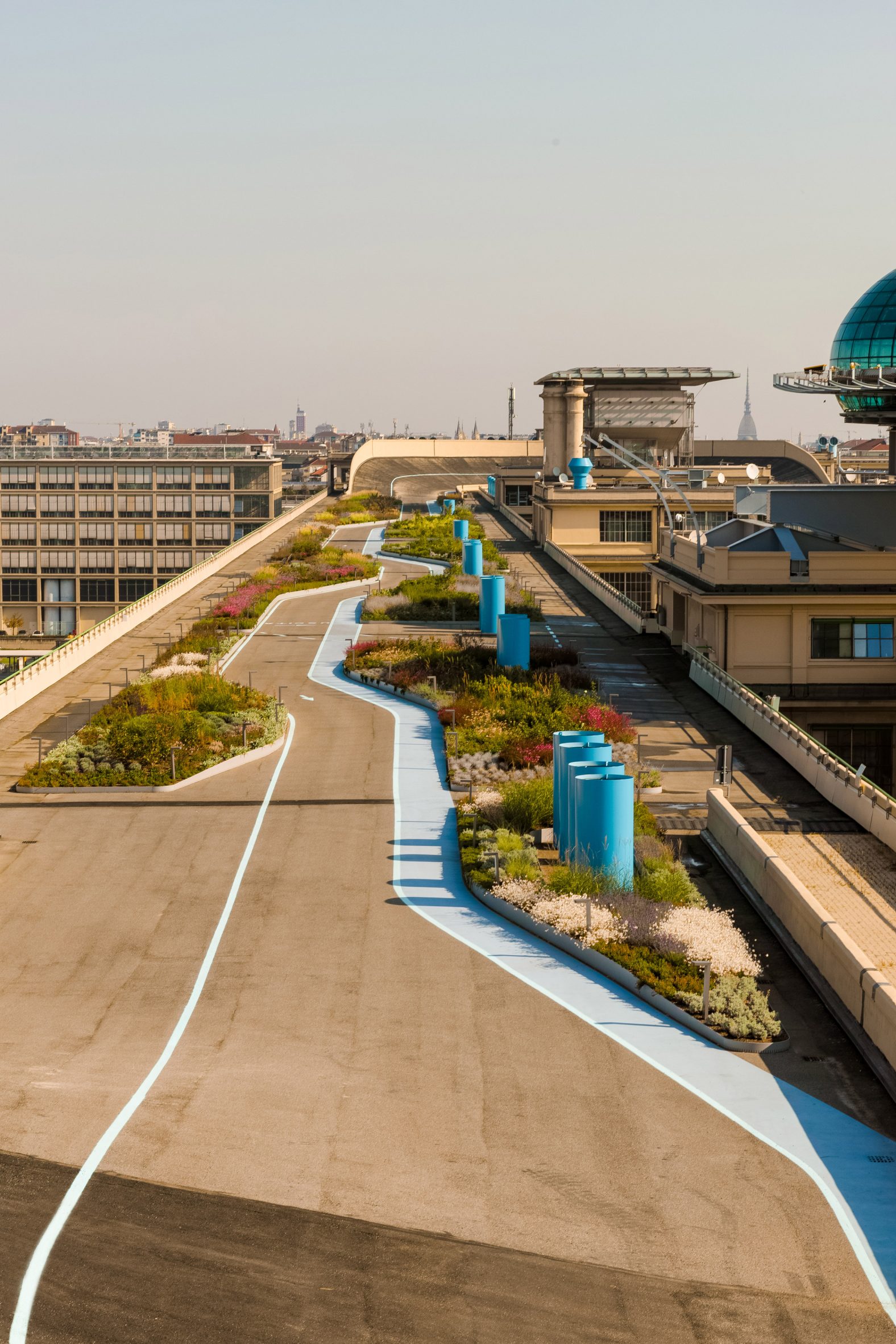The image captures an outdoor rooftop scene atop a large apartment building, high above the city streets and surrounded by towering skyscrapers. The rooftop has been thoughtfully converted into a green oasis with various gardens, featuring plantings of shrubs and colorful flowers in hues of white, red, and green. Blue cylindrical objects, possibly solar lights, are interspersed among the plant beds, with clusters of them visible both in the foreground and background. A striking blue path, which may serve as a bike lane or walkway, stretches from the right side of the image toward the back, bordered by small green spaces. The entire arrangement gives the impression of an elevated street or mini racetrack amidst a vibrant urban landscape.